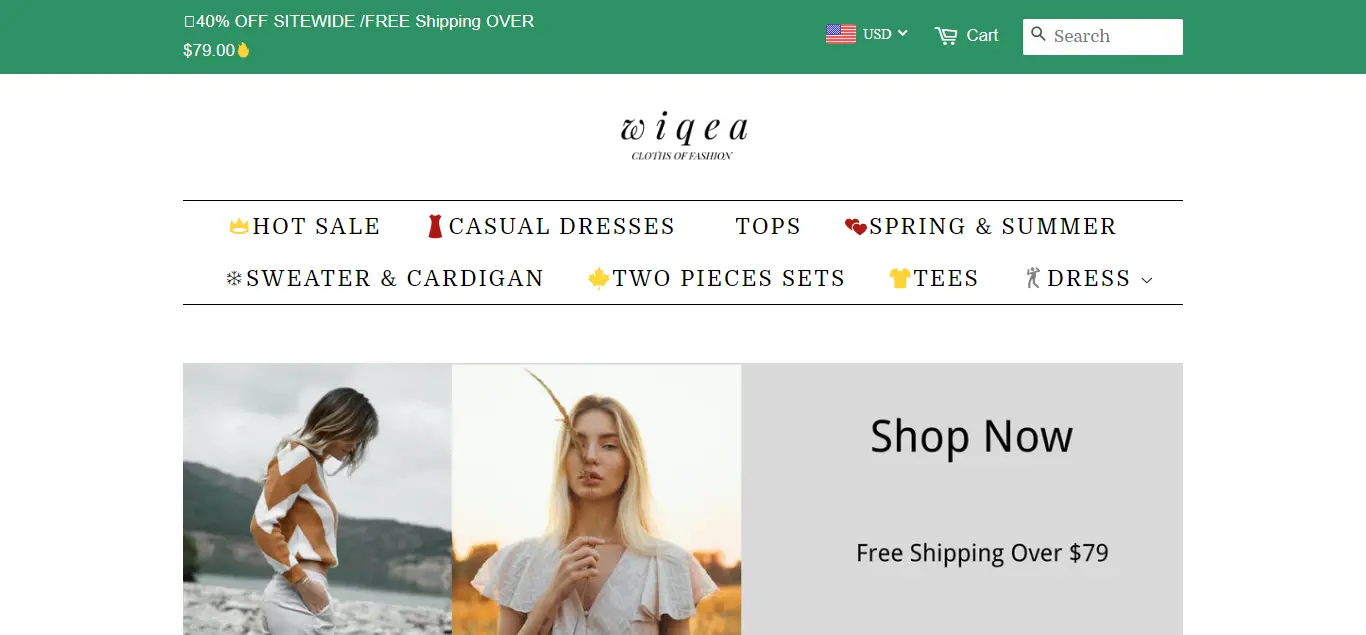The website features a predominantly white background with a striking green border at the top. Within the green border, in bold white font, a promotion reads: "40% off site-wide, free shipping over $79." To the right, an image of the American flag is displayed next to a dropdown menu labeled "USD," along with a shopping cart icon accompanied by the word "Cart," and a search box.

Directly beneath this border, a centered tagline on the white background reads: "WIKEA Clothes of Fashion." Below this, a dual-line box spans most of the screen, featuring a yellow crown icon and a bold "Hot Sale" announcement in black font. 

Within this section are various segments: 
1. A vibrant image of a red dress, labeled "Casual Dresses."
2. A segment for "Tops," named in black font.
3. An icon with two hearts, labeled "Spring and Summer."
4. An image of a snowflake, accompanied by the words "Sweater and Cardigan."
5. An icon of a yellow maple leaf, next to "Two-Piece Sets."
6. A yellow t-shirt image, labeled "Tees" in black font.
7. An icon of a person dancing, labeled "Dress," alongside a drop-down arrow.

Towards the bottom, there are two cropped images of different women placed side-by-side. Beneath these images, a gray box contains the text: "Shop Now, Free Shipping Over $79," centered within the box.